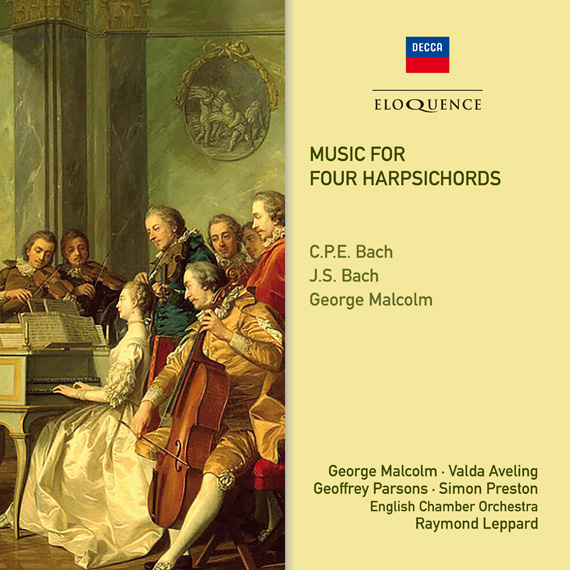The image appears to be an album cover for classical music. On the left side, there's an intricately detailed painting depicting a Renaissance-era scene set in a green-walled room. A woman, wearing an off-white, long-sleeved gown with her hair braided and styled in a ponytail, is seated at a white piano. Around her, half a dozen men clad in period attire of brown, green, and red are either playing violins and cellos or admiringly looking on. Above the woman, there's an additional painting featuring cherubic angels. 

On the right side, against an off-white background with a dark eggshell hue, the text reads "DECCA" at the top within a blue rectangle, followed by a black line and the word "eloquence" in black. Below this, it states "Music for Four Harpsichords," naming C.P.E. Bach, J.S. Bach, and George Malcolm as composers. Further down, the names George Malcolm, Valda Aveling, Geoffrey Parsons, Simon Preston, the English Chamber Orchestra, and Raymond Leppard are listed. The overall composition suggests a sophisticated classical music album, emphasizing its connection to the works of the Bachs and the participation of renowned musicians and orchestras.